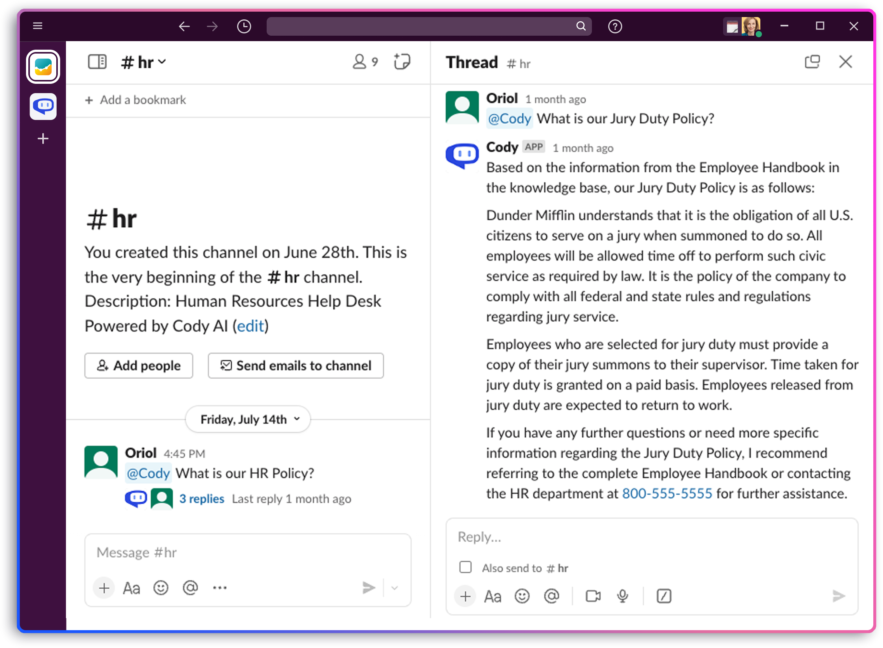The screen displays a communication from the Human Resources department within an in-house system. The overall visual theme includes a faint border gradient transitioning from purple in the top-left corner to blue, then circling back to purple at the bottom, and shifting to a bright pink on the top-right. This gradient encloses the predominantly white background of the interface. 

The top of the screen features a very dark purple bar, with a lighter shade of dark purple along the left side. In the left-side purple bar, there are two small icons: a blue speech bubble with eyes and a graph featuring yellow and blue segments.

The highlighted text reads: 
"#HR. You created this channel on June 28th. This is the very beginning of the #HR channel description. Human Resources help is powered by Kodi AI. You can edit that."

Below this introduction, there is a post from Aureole with the query: "What is our HR policy?" Subsequently, a threaded conversation is displayed wherein Aureole inquires about the jury duty policy. Kodi AI responds with detailed information from the employee handbook, stating:

"Dunder Mifflin understands that it is the obligation of all US citizens to serve on a jury when summoned. All employees are granted time off to fulfill this civil service as required by law. The company complies with all federal and state regulations regarding jury service. Employees selected for jury duty must provide a copy of the jury summons to their supervisor. The time taken for jury duty is paid. Employees released from jury duty are expected to return to work. For further inquiries or more specific information regarding the jury duty policy, refer to the complete employee handbook or contact the HR department at 800-555-5555 for assistance."

This detailed interaction underscores the company’s policy on jury duty and ensures compliance with legal obligations while providing necessary support to employees.